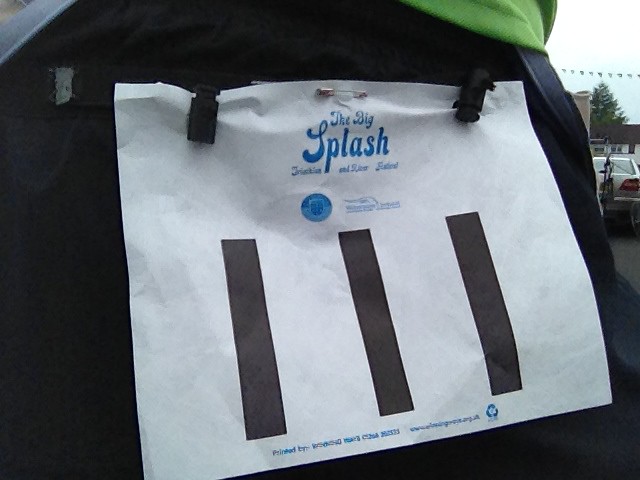The photograph is taken outdoors in a parking lot. In the upper right corner, a strip of the white sky is visible above a car, possibly a Volvo, with a bicycle attached to its rear. A neighboring tree rises from the background. Dominating the frame, approximately 90-95% of the image captures the back of a person wearing a dark, possibly black or navy blue, jacket with a green hood. Affixed to this apparel, via two small clips and a safety pin at the top, is a piece of paper. The paper displays the words "The Big Splash" in prominent blue letters at the top, followed by smaller, unreadable blue font. Additionally, three thick black lines run vertically from top to bottom underneath the title. Despite the extensive text and design details mentioned below the black lines, they are indiscernible in the photograph.